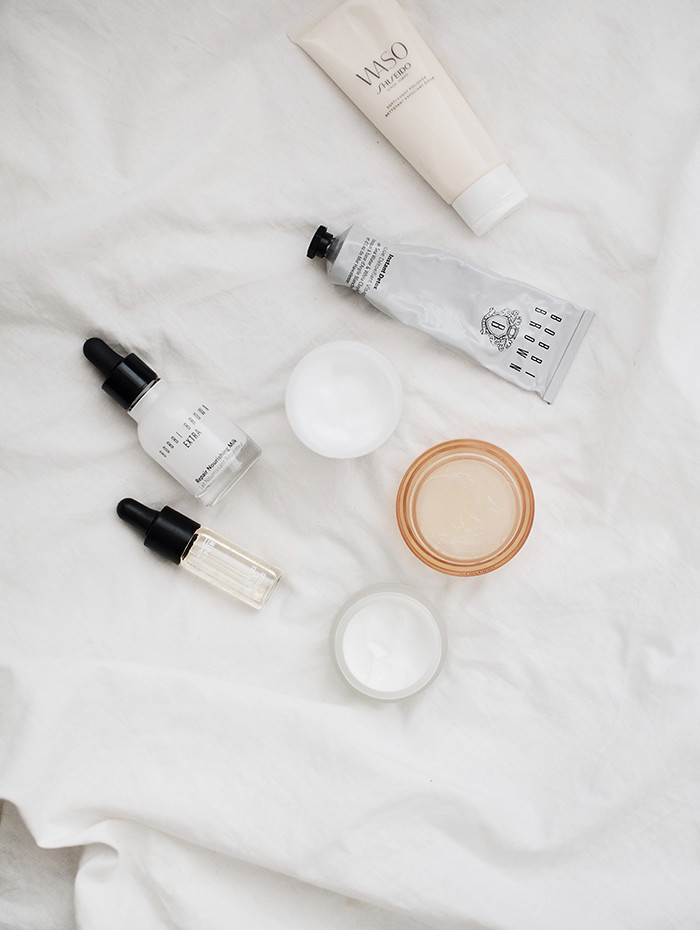The image showcases a close-up view of seven skincare and body care products meticulously arranged on a white linen sheet. Each item is distinct and adds to the composition of the photograph.

On the top right, there is a slender three-ounce tube of "Wasso Shiseido," featuring a white cap and a beige-toned base. Below it is a white tube from Bobbi Brown, which appears to contain an ointment. This tube is notable for its white body and black cap.

Next to them is a bottle labeled "Bobbi Brown Extra," resembling the size and shape of a nail polish bottle. This item has a white, semi-transparent glass outer casing with a black top. Adjacent to this is a slim, syringe-like bottle designed to dispense droplets, containing a white liquid and sealed with a black cap.

Completing the collection are three circular, disc-shaped containers, potentially used for storing creams or moisturizers for facial care. All seven products are neatly placed on the white linen sheet, providing a clean and organized representation of body care essentials.